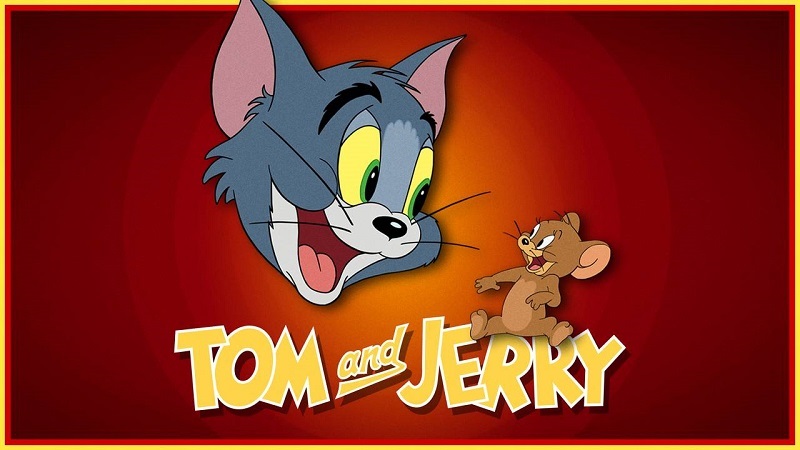The image is a vibrant cartoon opening for Tom and Jerry, set against a gradient red background that transitions to a lighter, orangey center. The text "Tom and Jerry" is prominently displayed at the bottom in bold, bright yellow uppercase letters with white borders, while the word "and" is in matching yellow lowercase letters. Dominating the center of the image, Tom, the cat, features a gray face with pink ears, yellow eyes with green irises, and a white snout accented by a pink tongue and red mouth. Tom's expression is one of cheerful curiosity as he gazes down at Jerry, the mouse, positioned to his right. Jerry is depicted as a brown mouse with a lighter brown chest and large, expressive eyes. Both characters are smiling, creating a lively and engaging scene typical of the beloved cartoon series.